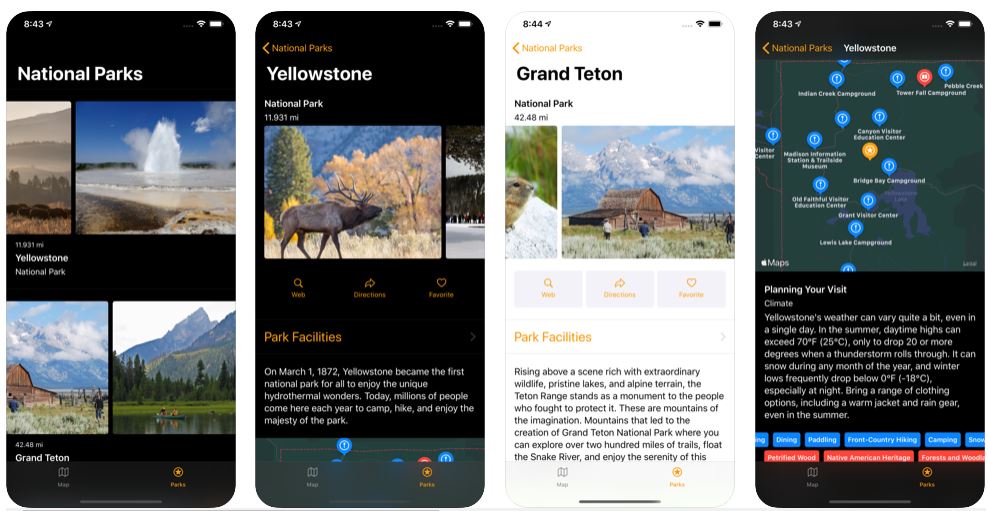The image consists of four neatly arranged screenshots from an Apple iPhone, with two screenshots placed side-by-side on the left and two on the right.

1. The first screenshot on the far left features a selection screen with a black background, showing images of various national parks. Prominently displayed parks include Yellowstone and Grand Teton, with accompanying scenic photos representing each park.
   
2. The second screenshot to its right is a detailed view of the Yellowstone National Park section within an app. At the top, it features a "National Parks" tab with a back button. Below, the word "Yellowstone" is displayed prominently, along with a partial image of a moose. Additional park facilities information and a map are visible lower in the frame, suggesting there is more content to explore by scrolling.

3. The third screenshot depicts similar information for Grand Teton National Park. This screen also includes thumbnail images and descriptive text about the park's attractions and facilities.

4. The screenshot on the far right displays a detailed map of Yellowstone National Park, highlighting various points of interest and visitor locations within the park. Below the map, more information is provided, presumably offering insights and navigation tips for visitors.

Together, these screenshots provide a comprehensive overview of a mobile app that offers valuable information and visual guides to some of the most prominent national parks in the United States.